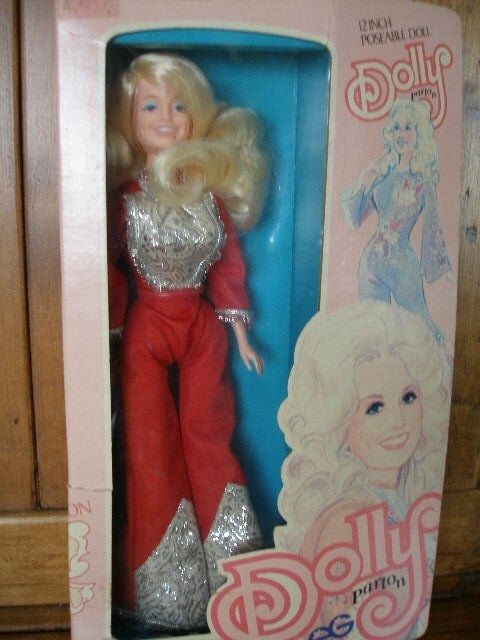The image captures a toy doll still encased in its packaging, prominently displayed against a dark plank wood surface, likely leaning against a cabinet or wall. The doll is modeled after the famous country singer Dolly Parton and is housed in a pink box. This box features a clear window on the left, showcasing the doll, while the right side contains informative text. The packaging reads "12 inch posable doll, Dolly Parton" and includes artistic renderings of Dolly Parton, highlighting her iconic curly blonde hair. The doll itself is centered in the image, occupying the entirety of the frame, and is dressed in a striking red jumpsuit adorned with silver and white embellishments. The various colors in the image are vivid, with different shades of pinks, reds, silvers, and the doll's blondish hair standing out against the darker wooden background.